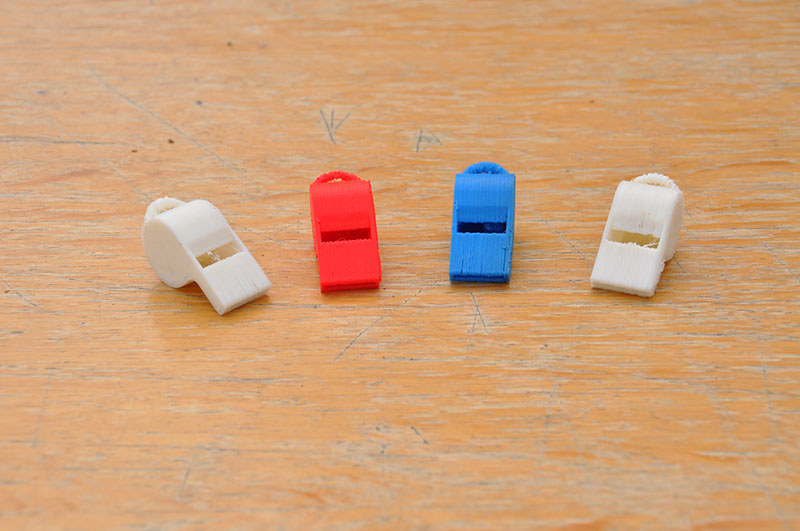This detailed color photograph captures four small plastic whistles arranged in a row across the middle of a light brown wood grain table. The table’s surface is noticeably worn and faded, featuring grayish spots of discoloration and random blue ink marks, as though someone had doodled on it with a pen. The wood grain pattern runs horizontally from left to right. 

The whistles, each with a small handle on top, have a rounded back and a slender mouthpiece. They feature a small rectangular hole near the mouthpiece for producing sound. From left to right, the first whistle is white and is slightly turned toward the bottom left corner. The second whistle is straight and red, followed by another straight blue whistle. The final whistle on the far right is white and slightly turned toward the top right corner. The combination of these brightly colored whistles against the dingy table adds a striking contrast to the image.